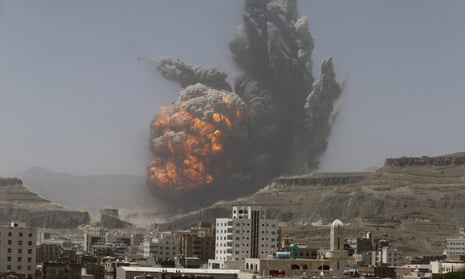The photograph captures a dramatic outdoor scene in a deserted, mountainous, and quarry-like landscape. Dominating the image is a massive explosion, characterized by a large fireball surrounded by thick, dark smoke that ascends into the blue sky, creating a towering plume. In the background, there are expansive, rocky, grayish mountains with no vegetation, reinforcing the desolate setting. In the lower portion of the image, particularly on the left side, stand a cluster of city buildings, including several smaller structures and taller, high-rise concrete buildings with numerous windows. The explosion's fiery core, displaying vibrant orange and red flames, contrasts sharply with the surrounding gray smoke, which hazes the entire skyline and underscores the scale of the blast reaching high into the atmosphere behind the cityscape.